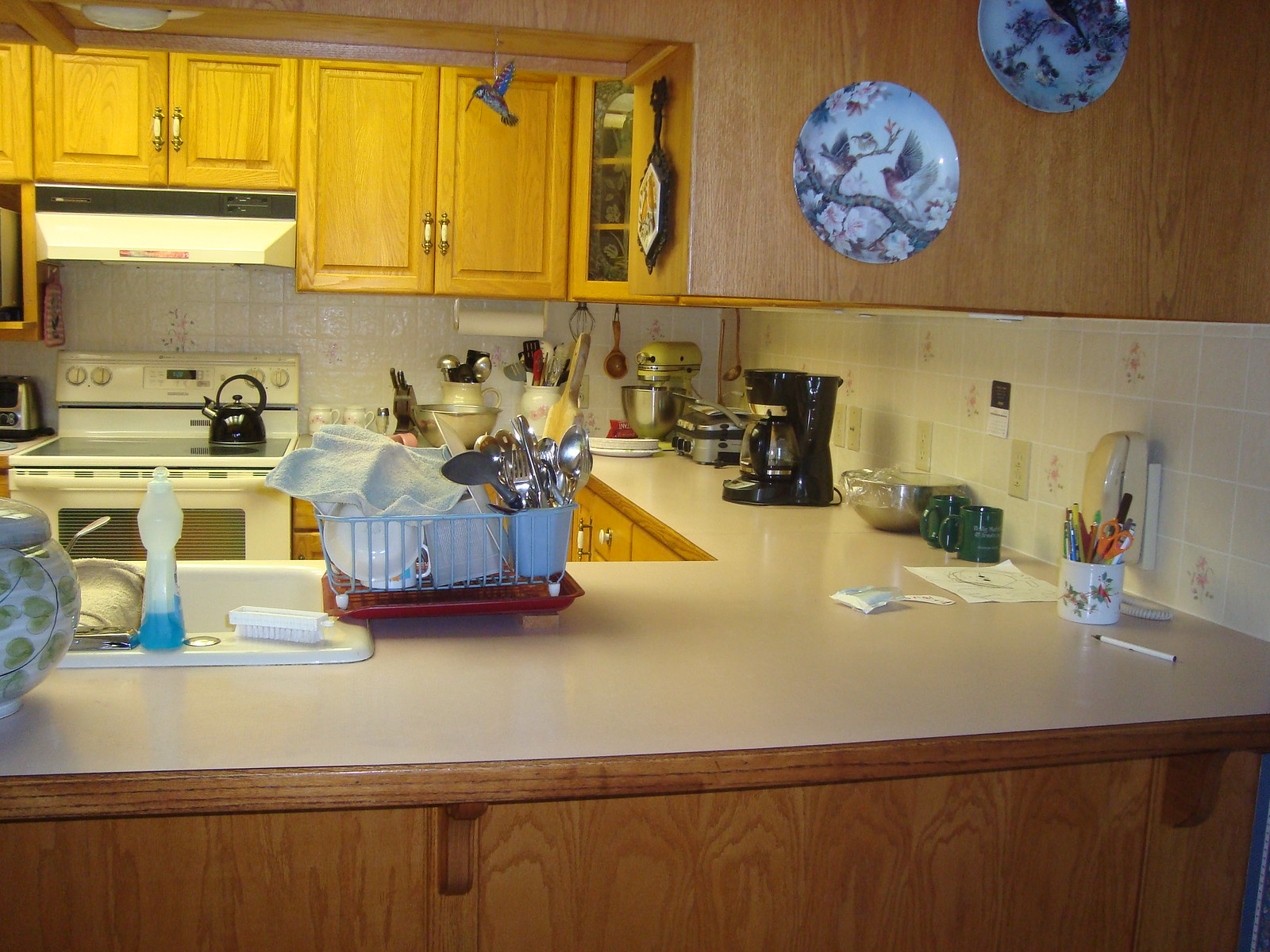The image depicts a kitchen scene characterized by its brown cabinetry and warm overhead lighting. A corner cabinet with a glass front houses a variety of items, providing a peek inside. On the wall above another cupboard, a delicate blue hummingbird ornament adds a touch of whimsy. Opposite this, a trivet and two blue plates, adorned with bird and tree motifs, decorate the wall.

The countertop is brimming with everyday kitchen essentials: a mug filled with pens, pencils, and scissors; two green mugs; a silver bowl covered with plastic wrap; and a coffee maker. Adjacent to these, a waffle maker sits alongside a stand-up mixer equipped with a silver bowl, and there are multiple containers filled with spatulas and spoons. A dish drainer in blue, resting on a red tray, contains an assortment of silverware. The teapot is positioned on the stove, next to a knife block bristling with knives.

By the sink, a scrub brush and a bottle of blue dish liquid are visible, with a white and green ginger jar completing the scene. This kitchen snapshot captures a blend of practicality and everyday charm, illustrating a well-used and well-loved space.